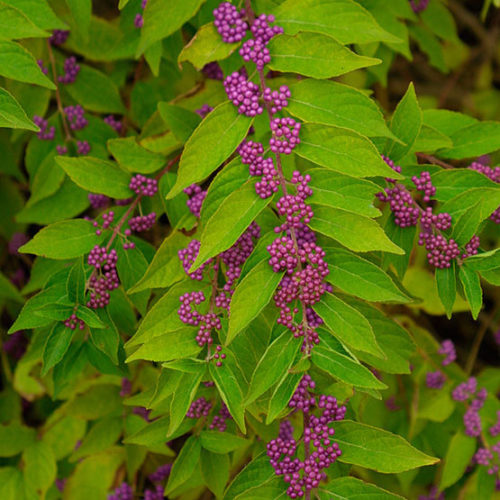This photograph is a detailed close-up of a lush, vibrant shrub adorned with clusters of tiny, bright purple beauty berries. The shrub's abundant green leaves stretch out horizontally and appear healthy and vibrant. Vertically hanging from stems, the purple berries resemble miniature pomegranates or blueberries, adding striking color contrast against the deep green foliage. The branches are long and filled with these vivid purplish-pinkish clusters. The background contains slightly blurred multiple shrubs, each featuring a single stem with beauty berries hanging down. Some brown branches are visible in the background, adding depth to the image. Overall, the image captures the dense arrangement of purple berries and green leaves, emphasizing the natural beauty and rich colors of the plant.